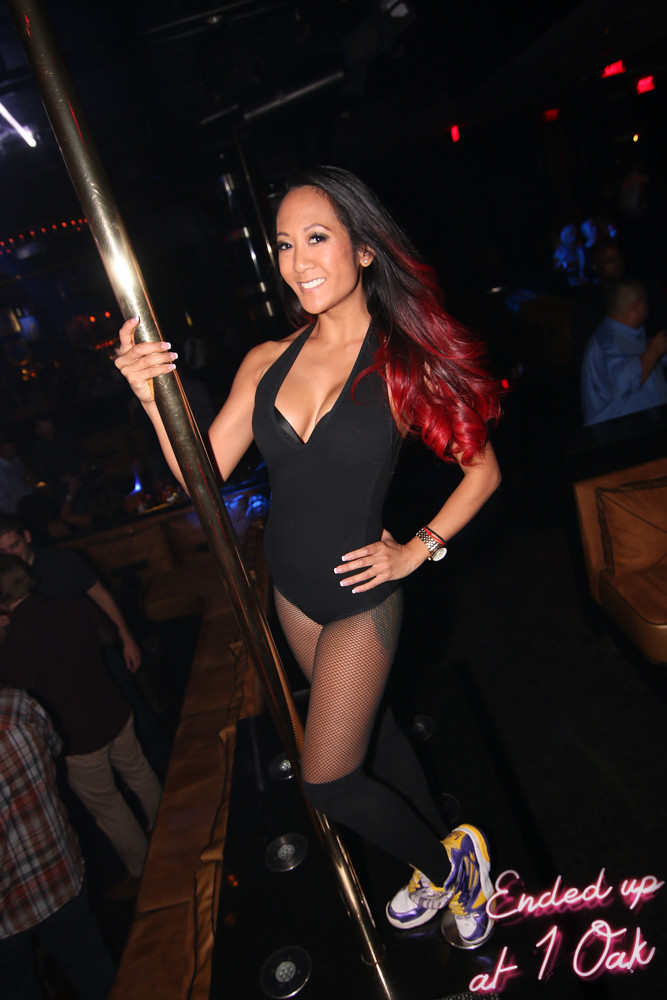The picture captures a youthful and attractive Asian woman standing confidently on a black stage at what appears to be a bar or club called "One Oak," as indicated by the bright pink LED text in the bottom corner of the image, although it's slightly tilted counterclockwise. She is artistically posed with her right hand twirled elegantly around a pole and her left hand resting on her hip. The woman is dressed in a plunging black unitard that highlights her bosom, complemented by black stockings and knee-high black socks. Her unique hairstyle features long, coiled black hair with striking red ends cascading down to her chest. She sports vibrant orange, white, and black sneakers. In the background, a dimly lit area can be seen, including a brown chair to the right and various spectators, some identifiable by the legs of individuals on the left and a person in a plaid shirt. The ambiance suggests she's preparing for a gymnastic or dance performance, as she stands elevated, possibly on a counter or podium, ready to showcase her skills on the pole.